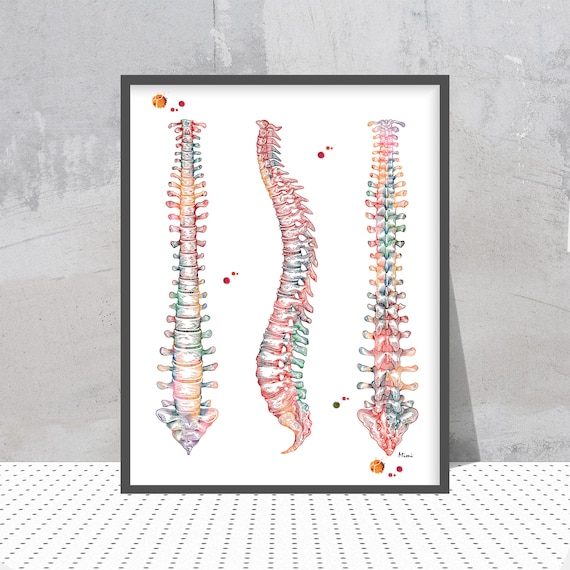The image features a monochromatic, textured gray concrete wall as the backdrop, with a white floor speckled with uniform black dots at the bottom. Propped up against the wall is a singular, black-framed picture which draws immediate attention. The picture itself displays three multicolored views of the human spine, presenting it from different angles such as the front, side, and back. The spine illustrations showcase a full spectrum of colors, including vibrant reds, greens, blues, and oranges, capturing the intricate details of the bone structure and discs. Scattered throughout the image within the frame are clusters of small red dots, adding an interesting visual contrast. There is also a line of small black text at the bottom of the picture, though it is not clearly legible.